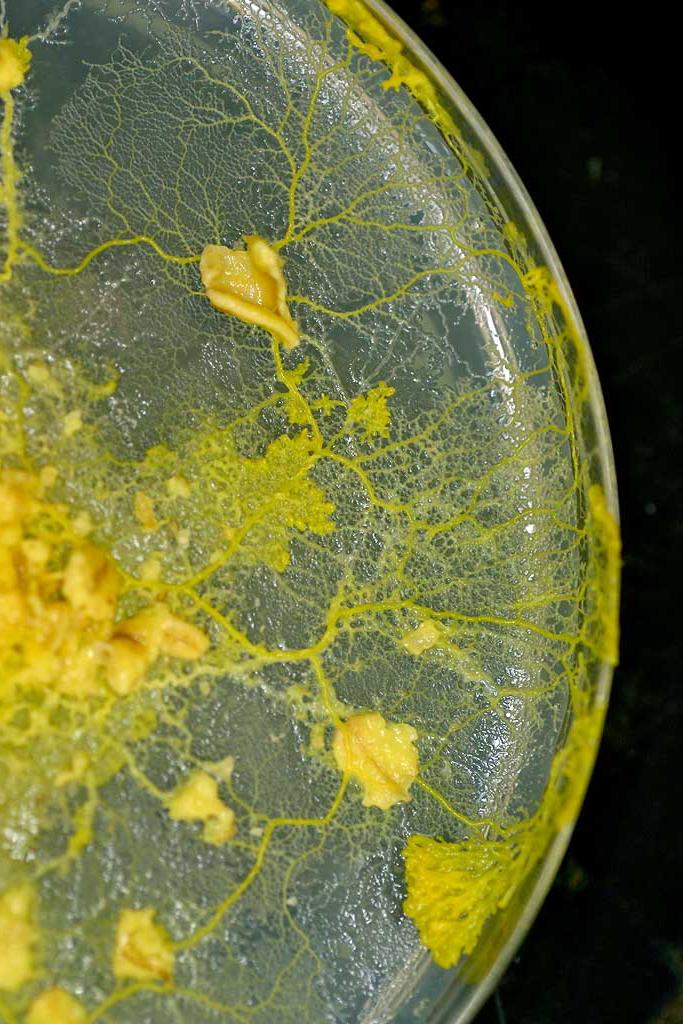This photograph showcases a Petri dish containing plasmodial slime mold cultured on an agar base, which serves as the growth medium. The mold, a light green hue, displays a sprawling, intricate network reminiscent of branching tentacles radiating outward. At the center of the dish, the mold appears to have thickened and slightly piled up, forming curled edges and overlapping layers that resemble delicate, curled leaves. Moving towards the edges of the Petri dish, the slime mold's structure becomes more slender and web-like, evoking the silhouette of a bare tree in winter. This detailed image captures the unique morphology and expansion pattern of plasmodial slime mold on agar.